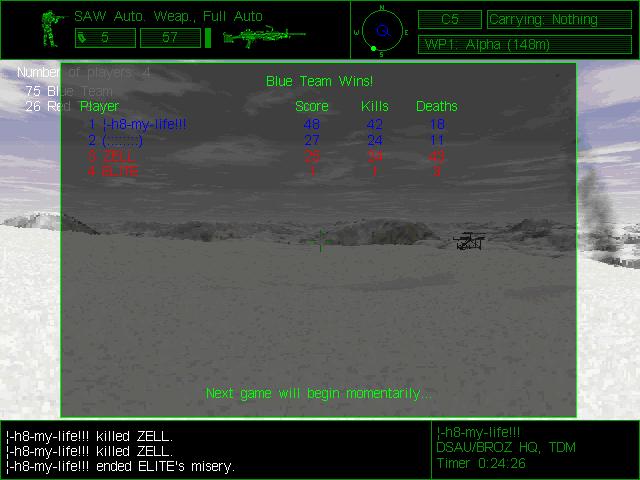This is a screenshot from an older pre-2010 video game with a snowy, mountainous backdrop. The screen prominently displays a message in green text that reads "Blue team wins." Superimposed on the snowy scene, a grayish, semi-transparent overlay with a green border provides a detailed score summary: the player "hate my life" has a score of 48, with 42 kills and 18 deaths. In smaller, colored text, it shows players listed with their respective scores and kills in blue and red. The bottom of the screen is bordered by a black bar that recaps recent actions, with phrases like "hate my life killed Zell" and "hate my life ended elites misery" repeated. At the top, an icon of a green-outlined character holding a high-powered rifle is displayed, accompanied by the text "SAW auto weapon full-auto, five clips and 57 bullets in the current clip." To the right, a compass and a map indicator provide additional gameplay information. The words "Next game will begin momentarily" suggest the game is transitioning to a new round. A timestamp "TDM timer 0:24:26" is visible in the bottom right corner.